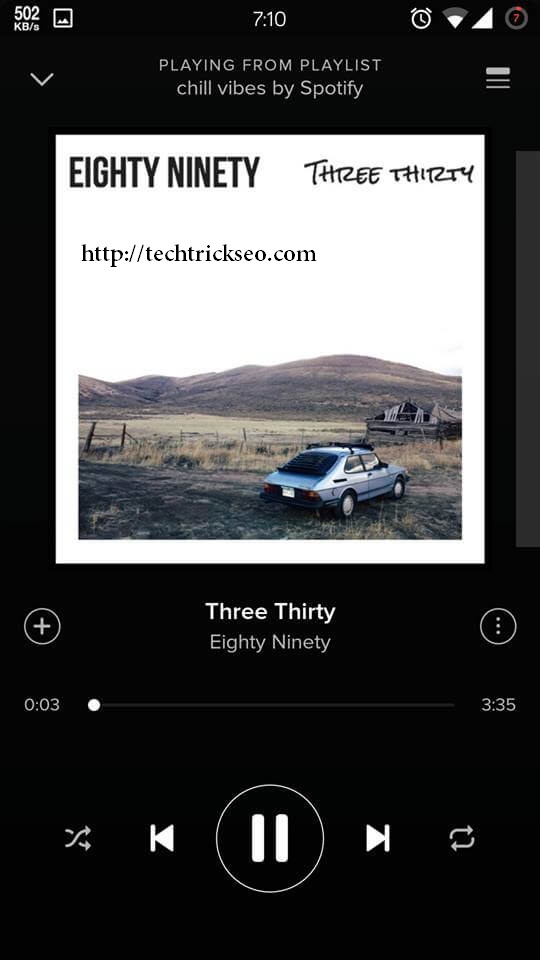This image, captured from a cell phone screen, prominently features a black background that accentuates a central white square. Within this square, there is a small, light blue, two-door car, which includes black plastic strips on the windshield and rear window. The car is parked in an isolated, hilly field with a dilapidated barn visible in the background.

The overlay on the image shows details from a music playlist titled "Chill Vibes by Spotify." At the top of the screen, "8090" is displayed in bold, capitalized black letters. To the right of this, handwritten in a casual script, is the number "330." 

A URL is also visible: "http://tech trickseo.com." The current song playing is "330" by 8090, and the playback status indicates the track is three seconds in, with the usual media control buttons (pause, fast forward, reverse) displayed underneath.

This well-composed snapshot blends elements of technology and serene landscape, providing a glimpse into a moment of auditory and visual retreat.